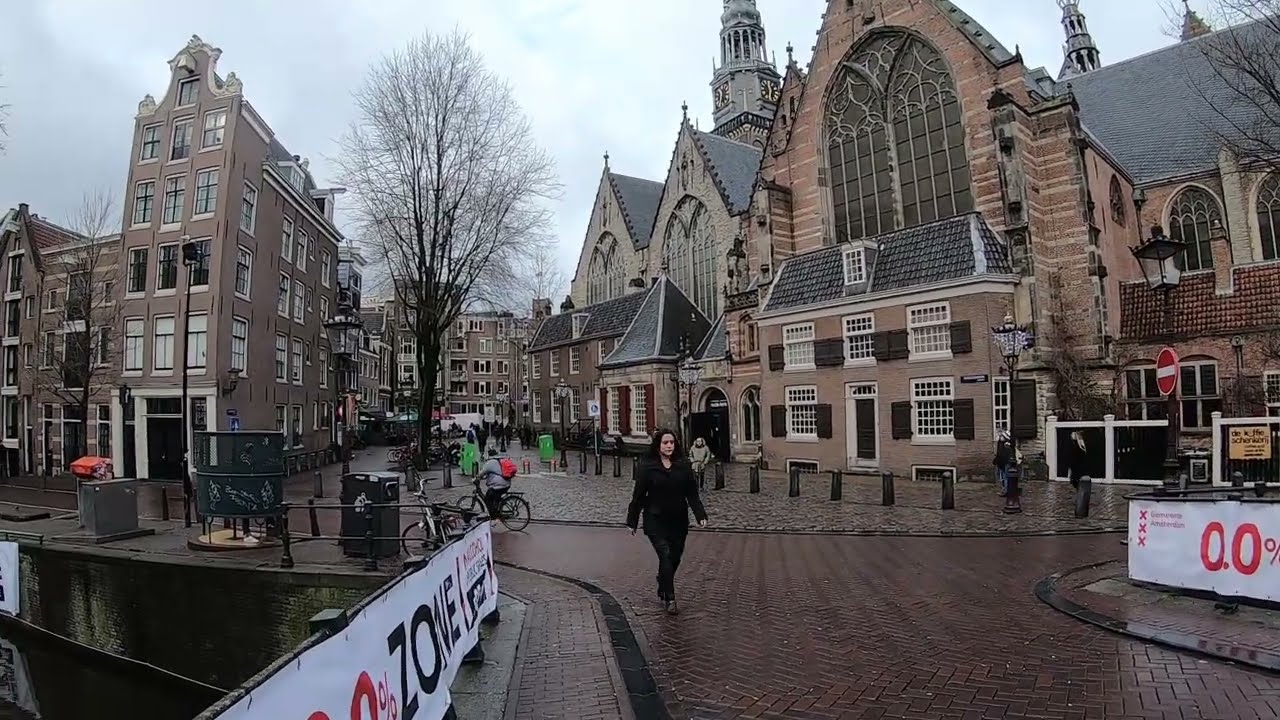The photograph captures a bustling town square set against a backdrop of eclectic buildings. On the right side, a row of gothic architectural structures with beige and gray facades, accented by white window trims and brown shutters, stands proudly. Among them is a potential clock tower, adding historical charm. On the left side, a more modernized building contrasts sharply with its older counterparts. The ground is a patchwork of red brick pathways and a central cobblestone area lined with cement poles in front of the buildings.

In the middle of this lively scene, a woman dressed entirely in black, with long dark hair, walks towards the camera, drawing attention due to her contrasting attire. The square is animated, with figures in the background, including an individual cycling through the paved walkway. To the left, a leafless tree and what appears to be an elevated wall with possible watermarks hinting at a nearby body of water add to the texture of the setting. The image is bathed in natural daylight, capturing a sky with whitish-gray clouds, indicating overcast weather. The glistening walkways suggest that the area might have experienced recent rainfall. Numbers reading "0.0%" are visible on the right side of the image, possibly a digital overlay. The overall scene offers a blend of historical architecture, modern elements, and daily life in a picturesque, tourist-friendly locale.